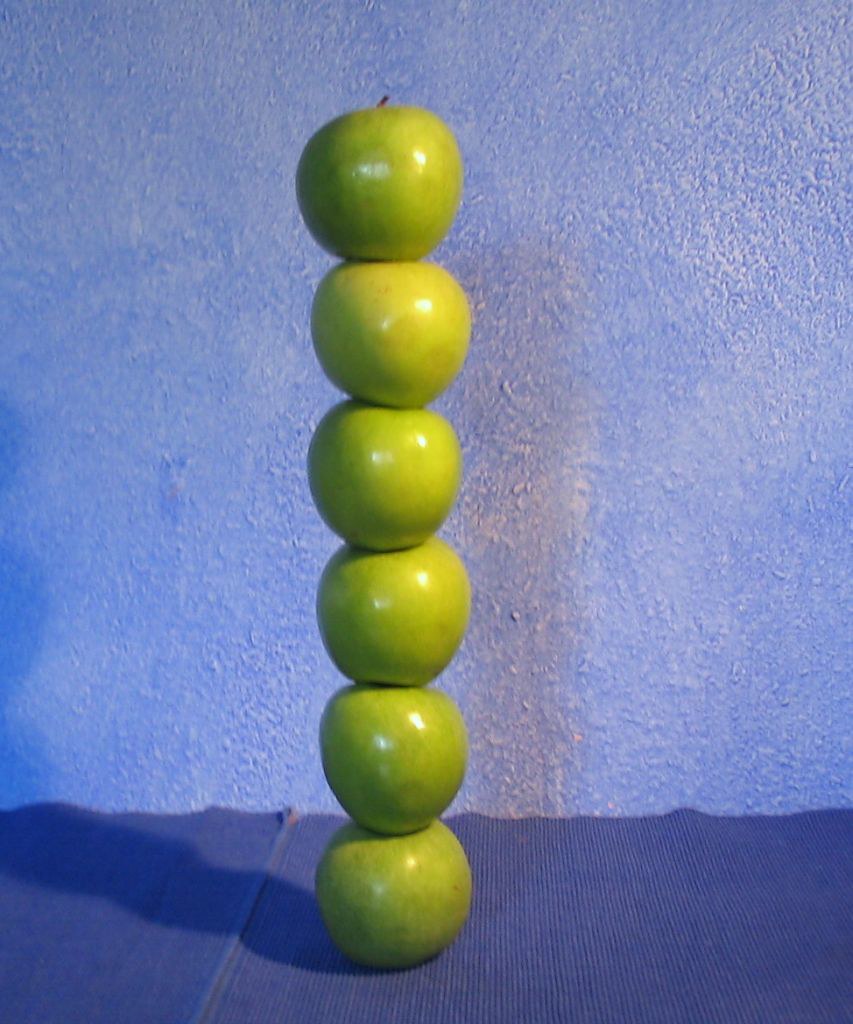This detailed photograph showcases a meticulously arranged stack of six vibrant green apples, balanced vertically in front of a blue stucco wall. The background is a predominantly blue surface with subtle white accents, while the base upon which the apples rest appears to be a darker blue material, possibly cloth or corduroy. Each apple looks ripe and in excellent condition, with a noticeable shine, particularly on the top right, suggesting a deliberate light source. The top apple displays its stem, whereas the stems of the lower apples are hidden, leading to speculation that they might be glued or skewered to maintain their perfect alignment. The careful arrangement is further highlighted by the shadows cast to the bottom left of the apples. The image lacks any people or text, focusing solely on the artful composition of the apples against the contrasting blue background.